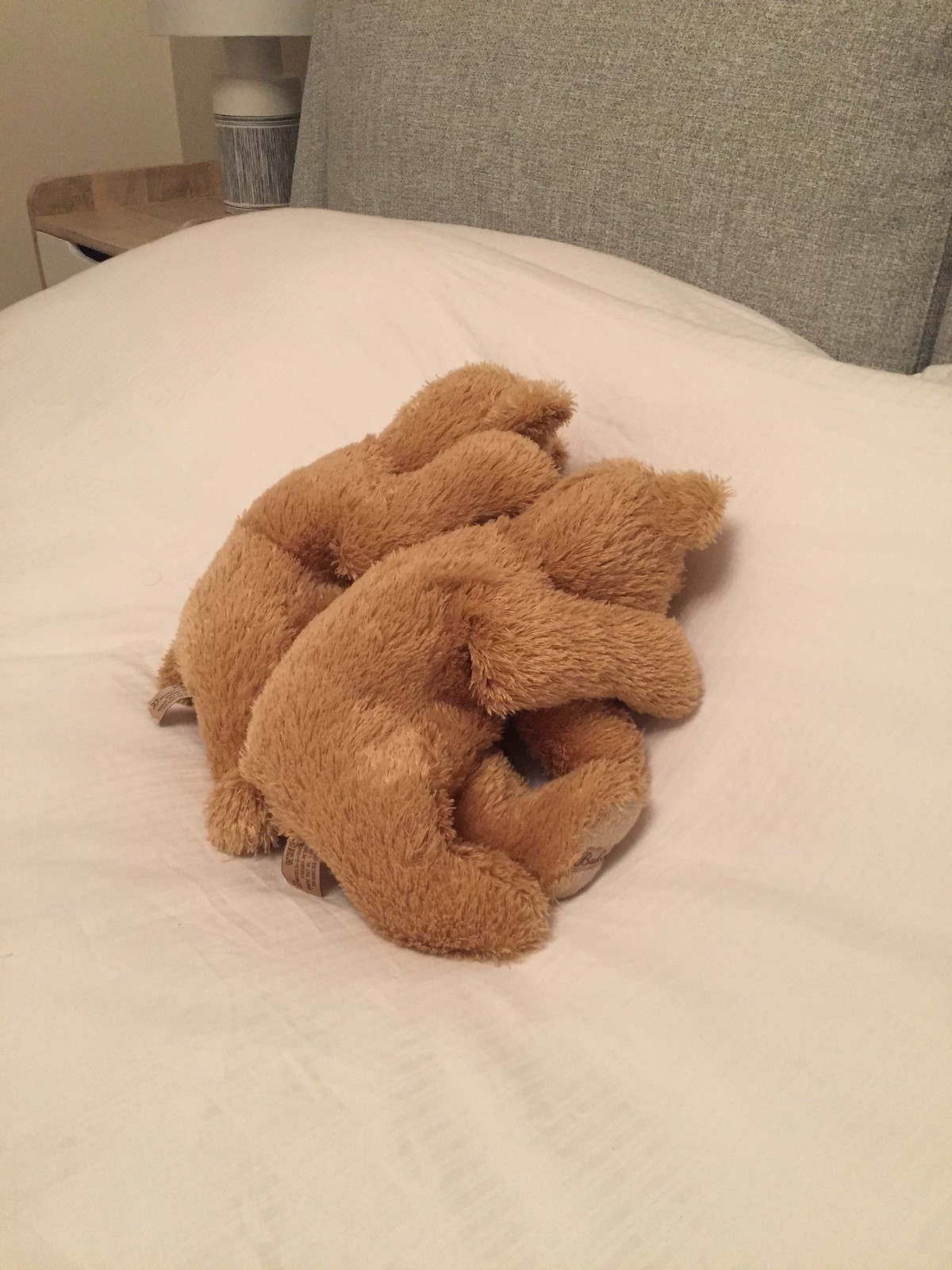This photograph captures a cozy and intimate scene of two brown teddy bears lying side by side on a bed. The bears appear to be in a cuddling position, with one bear spooning the other, both of them laying on their sides with their paws covering their faces, giving the impression that they are sleeping or perhaps crying. The plush bears have soft, tan fur, with lighter-colored fur on the bottom of their feet and curved ears. The bed is made with a white sheet and a cream-colored comforter, offering a soft, inviting look. At the top of the bed, against what seems like a headboard or cushion, is a gray linen pillow, enhancing the bed's modern and smart design. Beside the bed is a wooden nightstand featuring a blue and white ceramic lamp with a white lampshade and a gray pattern. The nightstand also has a white drawer beneath its wood-grain top. The overall atmosphere created by this arrangement is one of warmth and comfort, invoking a sense of gentle care and calmness.